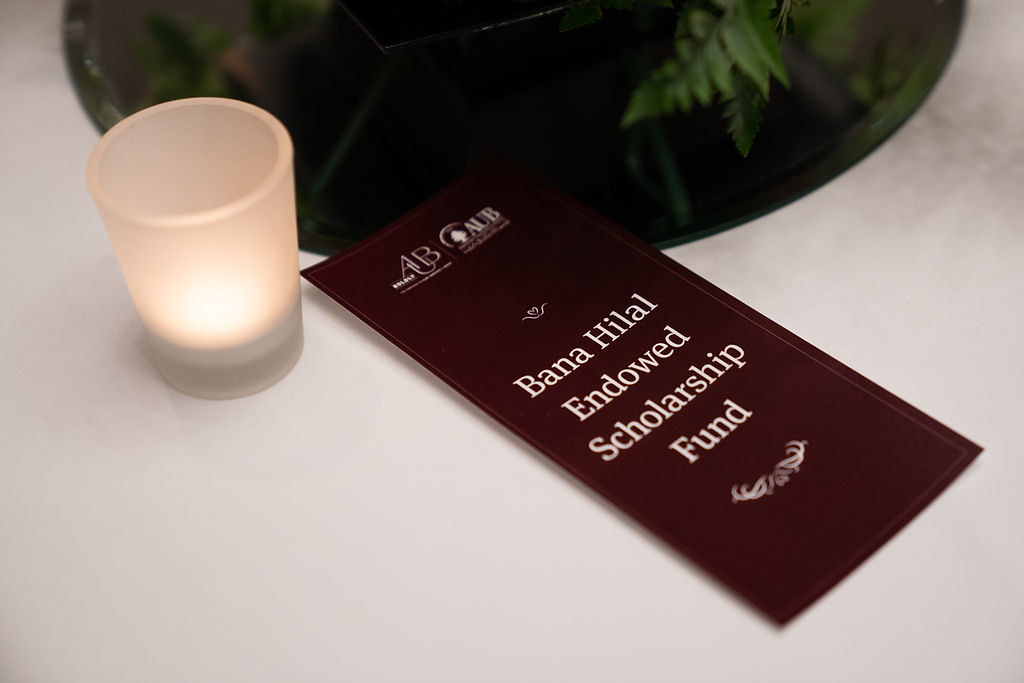The image showcases a diagonally placed dark brown brochure on a white table, prominently featuring white text that reads "BANNER HILLEL ENDOWED SCHOLARSHIP FUND" in four center-justified lines. Decorating the brochure are small scroll designs above and below the text, with two company logos at the top, albeit partially blurred. To the left of the brochure, there is a frosted white candle holder with a lit, well-used tea light candle. Behind the candle and the brochure, a tray with green plant leaves, casting a subtle shadow, adds a touch of nature. The entire arrangement rests on a white tablecloth, capturing a serene and thoughtful scene.